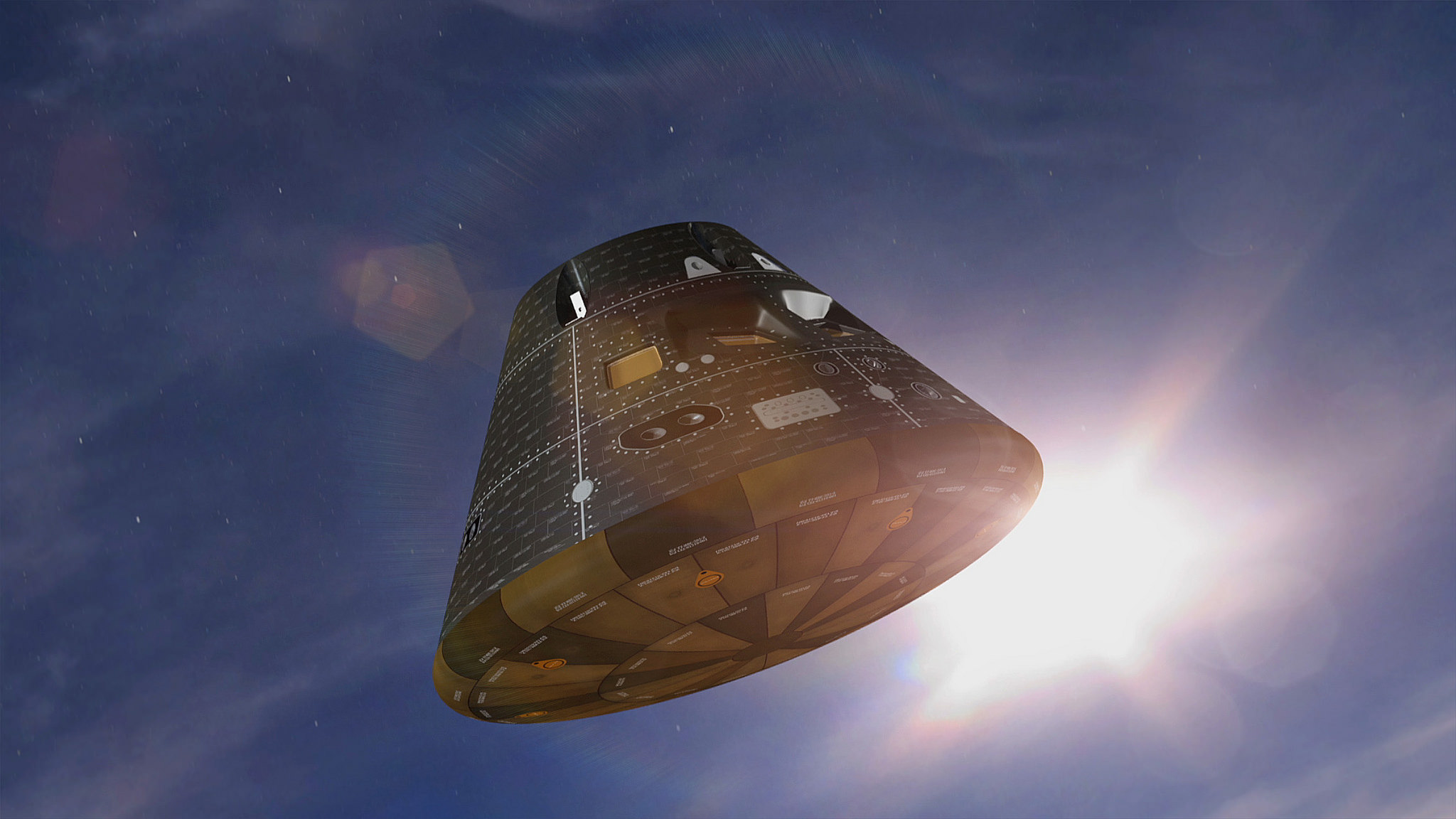The photograph captures a futuristic, oblong cylindrical satellite suspended in the deep blue sky with the sun faintly visible at the bottom right, casting a light that accentuates its size. The satellite, resembling a cone or volcano shape, features a wider base tapering to a narrower top. Its exterior consists of alternating sections of black and tan colors, with rings and layers at the bottom, likely made of some complex material. White lines delineate the structure, giving it a geometric, compartmentalized appearance adorned with several panels or "compartments", each with text or numbers that are not entirely legible. Noteworthy are the darker green, almost navy-colored windows positioned along the sides, suggesting an extraterrestrial or exploratory function. The three ascending sections of the satellite contain various graphs and measurement tools, highlighted by specific squares and dark spots, including two round circles on the bottom ring, enhancing its intricate and scientific design.